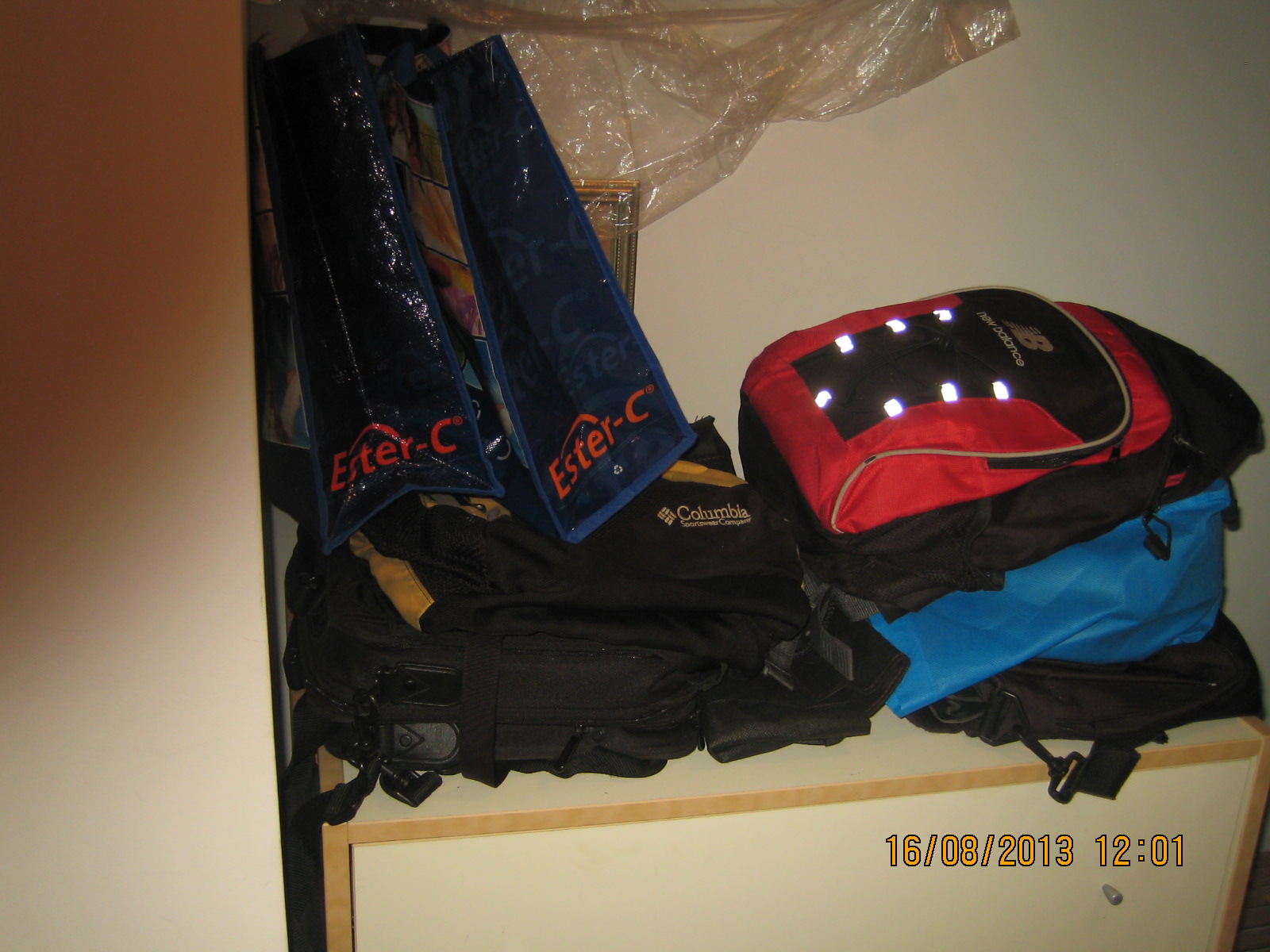In a storage area or closet with an off-white and tan-colored background, there is an arrangement of sporting equipment resting on a white dresser with brown trim. The dresser is situated within a cubby hole. On top of the dresser, there's a blue backpack with a red and black backpack placed on it. The red and black backpack has seven fluorescent lights protruding from it. To the left of these backpacks, there is another black backpack and a Columbia sports luggage case. Hanging from an unseen bar, possibly a garment bag, is a piece of clear dry-cleaning plastic. Additionally, there are two rectangular blue containers labeled “Esther C.” The photograph is dated August 16, 2013, with a timestamp of 12:01.